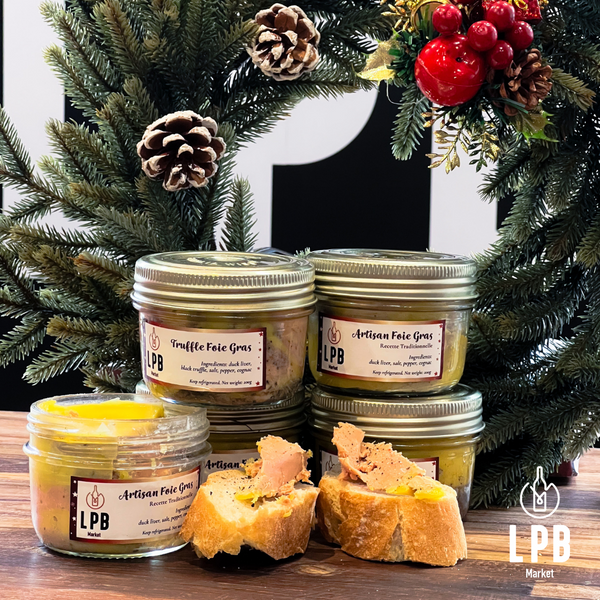This vertical rectangular photograph, likely an advertisement or product listing, features a festive Christmas scene centered around a selection of gourmet food items. In the background, a lush green Christmas wreath adorned with pine cones, grapes, cranapples, and ornaments adds a holiday touch. The foreground displays four or five mason jars labeled "Artisan Foie Gras," a delicacy made from fatty duck liver, sitting on a brown wooden table. One jar is open, revealing the yellowish-pink spread inside, which is also smeared on a couple of bread slices beside the jars. The jars and bread are set against a backdrop with partially obscured white-on-black text, likely part of the branding or marketing message, and the bottom left features "LPB Market" in large letters, indicating the source or retailer of these gourmet items. This image seems tailored for Christmas gifting, evoking both festive cheer and culinary sophistication.